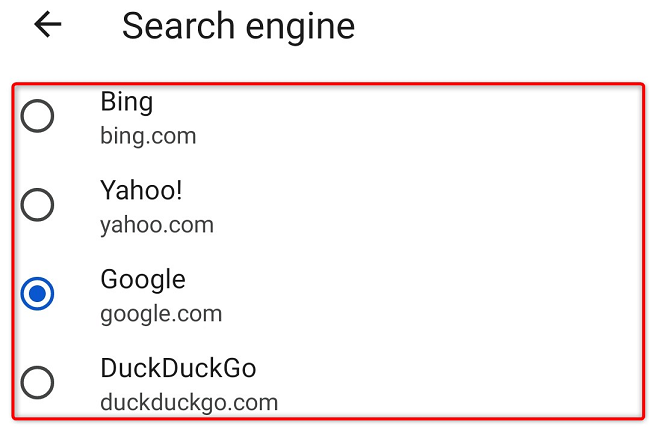The screenshot features a user interface for selecting a preferred search engine. The background is plain white and centrally displays the text "Search Engine" along with an arrow pointing to the left. Below this header, there are four options listed in sequence, each accompanied by a radio button that allows the user to make a selection:

1. **Bing** - represented by the URL "bingbing.com" enclosed in a red rectangular box, with an adjacent circle indicating the radio button.
2. **Yahoo** - denoted by the URL "yahoo.com" with a circle for the radio button.
3. **Google** - indicated by the URL "google.com", and this option is currently selected, as shown by a blue-highlighted circle next to it.
4. **DuckDuckGo** - shown with the URL "duckduckgo.com" and its respective radio button circle.

Once a search engine is selected, the corresponding radio button changes from gray to blue, signifying the active selection. The interface's simplicity is highlighted by its lack of additional text or default labels, maintaining a clean and uncluttered appearance.